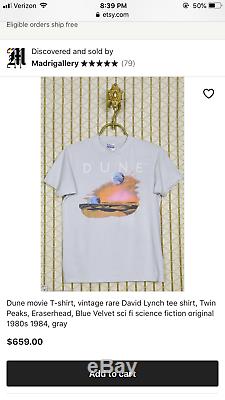A smartphone screen displays an eBay listing, although the top of the screen mistakenly shows the Etsy.com logo. The screen reveals it’s 8:39 PM on a Verizon phone, with the battery level at 50%. Text at the top indicates "Eligible orders ship free," alongside a stylish calligraphy "M" and the note "discovered and sold by Maddie Gallery," boasting a five-star rating based on 79 reviews.

The focus of the listing is a t-shirt hanging on a hanger. The shirt features the word "Dune" and an image of a dune. Descriptive text on the listing reads "Dune movie t-shirt vintage rare David Lynch t-shirt Twin Peaks Eraserhead Blue Velvet sci-fi fiction original 1980s 1984 gray." This rare vintage item is priced at $659.